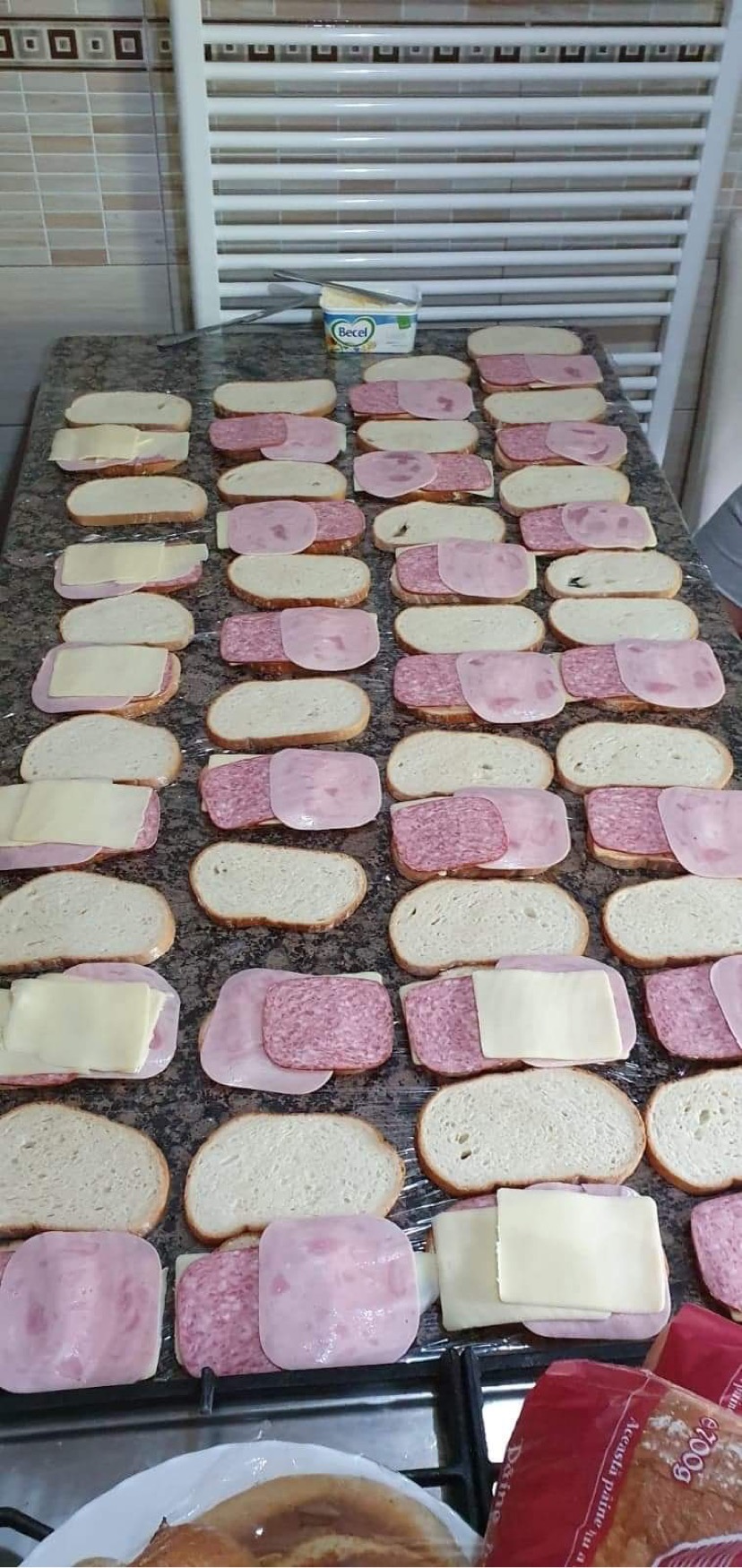The photograph captures an assembly line of open-faced sandwiches meticulously arranged on a black and brown marble countertop, which is detailed with darker splotches. Lining the counter, there are at least 24 sandwiches being prepared, with 48 pieces of white sandwich bread spread out in a grid formation of 4 rows across and 12 down. Each alternate row is topped with slices of white cheese—likely Swiss or provolone—alongside pink ham and more reddish-pink salami. Some sandwiches are merely bread, awaiting further assembly.

The backdrop features a beige and brown-tiled wall with square designs, and beneath it lies a strip of light-colored bricks tinged with shades of light red and blue. In front of the wall, there's some kind of grate or rack structure. At the edge of the counter in the bottom-right corner, part of a sandwich bag and a plate can be seen. Notably, there are two bread packages wrapped in red and clear plastic, and an opened tub of butter sits at one end of the counter, suggesting ongoing sandwich preparation. The meticulous layout and large number of sandwiches suggest this could be part of a large-scale effort, maybe for a school event or similar occasion.